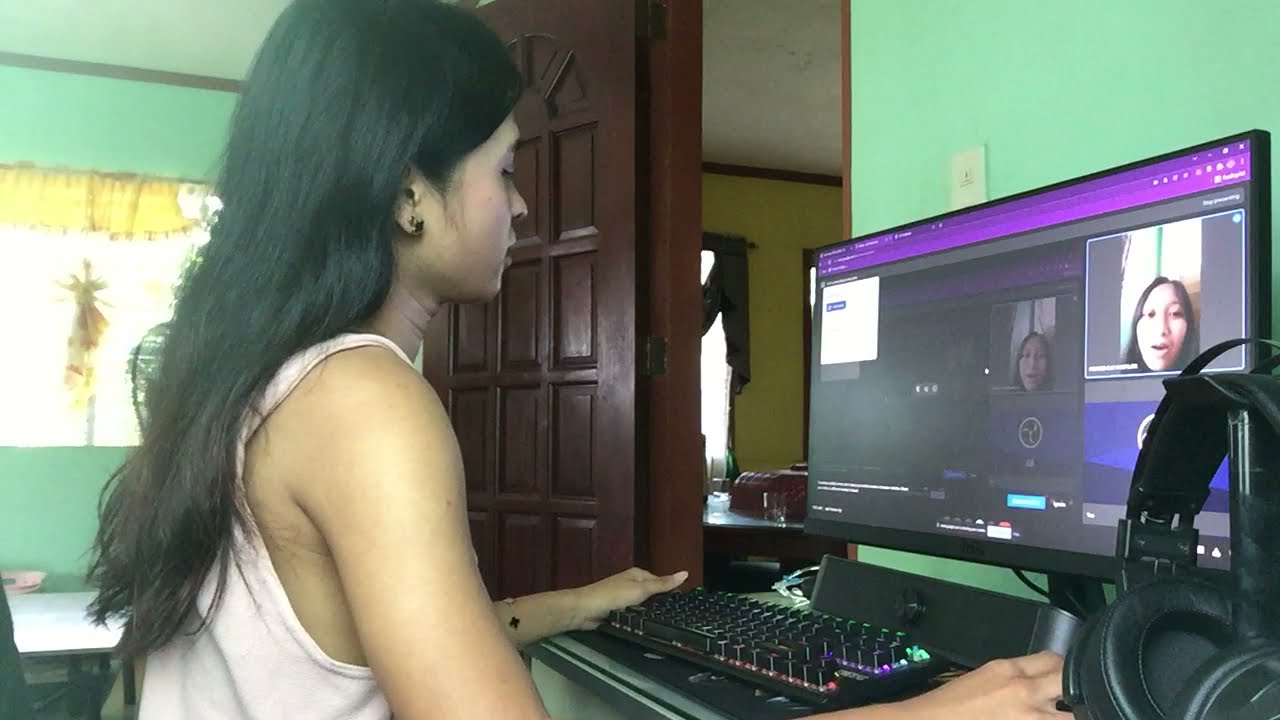In this photograph, we see a detailed interior setting featuring a woman engaged in a Zoom call. Positioned on the left side of the image, the woman, who appears to be of Indian descent with long black hair and darker skin, is shown in a side profile, intently looking at her computer monitor. She is wearing a white muscle shirt and her hands are resting on a table that holds a black keyboard and a desktop monitor. The monitor displays multiple faces in tiles, typical of a Zoom call interface.

The room's walls are painted light green, with a front wall featuring a window that lets in bright natural light. Adjacent to the green walls is a sturdy brown door with wooden cutouts, leading to another room with yellow walls. Above the door, a yellow valance curtain hangs, adding a touch of elegance and color contrast. In the bottom right corner of the image, we notice over-the-ear headphones placed on a stand. Overall, the scene captures a moment of virtual interaction amidst a well-lit and organized room.